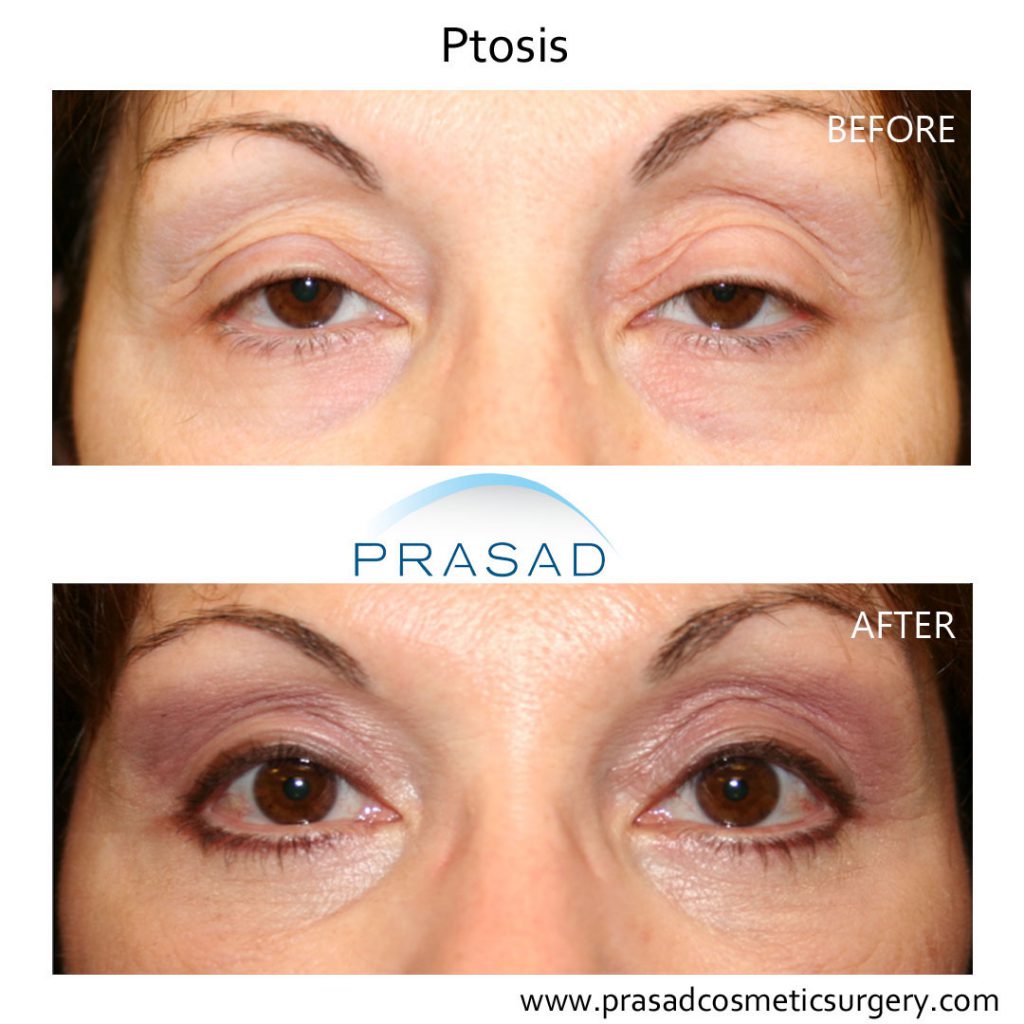The image is a detailed before-and-after comparison from Prasad Cosmetic Surgery, showcasing the results of an eye lift procedure for ptosis. The before photo, labeled "Ptosis," features a close-up of a woman's eyes, which appear markedly baggy and hooded, indicating droopy eyelids. In the contrasting after photo, positioned below and separated by the text "Prasad," her eyes look significantly less droopy and more vibrant, with an overall lifted appearance. The transformation highlights a notable enhancement in the eye area, potentially improving both aesthetics and vision. At the bottom of the image, the website www.prasadcosmeticsurgery.com is displayed, clearly indicating the provider of this cosmetic surgery service.